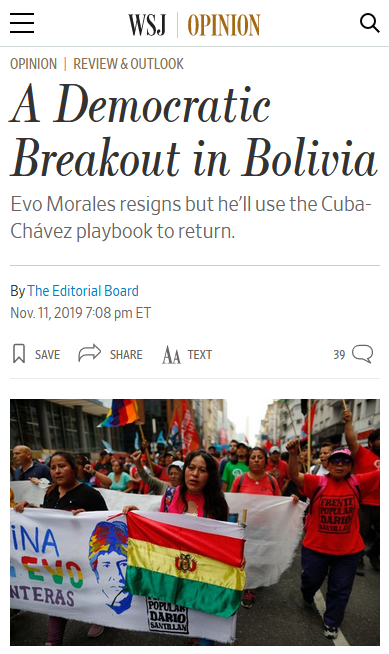This image is a screenshot from a Wall Street Journal article captured in portrait mode. 

- In the upper left-hand corner, three black lines are visible.
- The top center displays the Wall Street Journal logo, abbreviated as "WSJ".
- Below the logo, in brown capital letters, the word "OPINION" is prominently shown.
- The upper right-hand corner features a search icon.

A gray line separates this section from the main article content.

- The headline is written in all capital letters: "OPINION REVIEW & OUTLOOK".
- Below this, in cursive, the title reads: "A Democratic Breakout in Bolivia".
- The subtitle states: "Evo Morales resigns, but he'll use the Cubo Chavez playbook to return".
- Another gray line follows.

Authorship information is then provided:

- "By" followed by "The Editorial Board" in blue, indicating it’s a live link.
- The date and time formatted as "November 11, 2019, 7:08 PM Eastern Time".

The next row includes icons for saving, sharing, and adjusting text, followed by an icon indicating there are "39 comments".

- Another gray line appears.

The central image, cut off at the right-hand side where crediting should be, depicts a large crowd of people marching. They carry white banners with the words "Ina" and "Evo Popular" visible. Prominently featured is a red, yellow, and green Bolivian flag. The crowd appears to be mostly composed of individuals of South American descent.